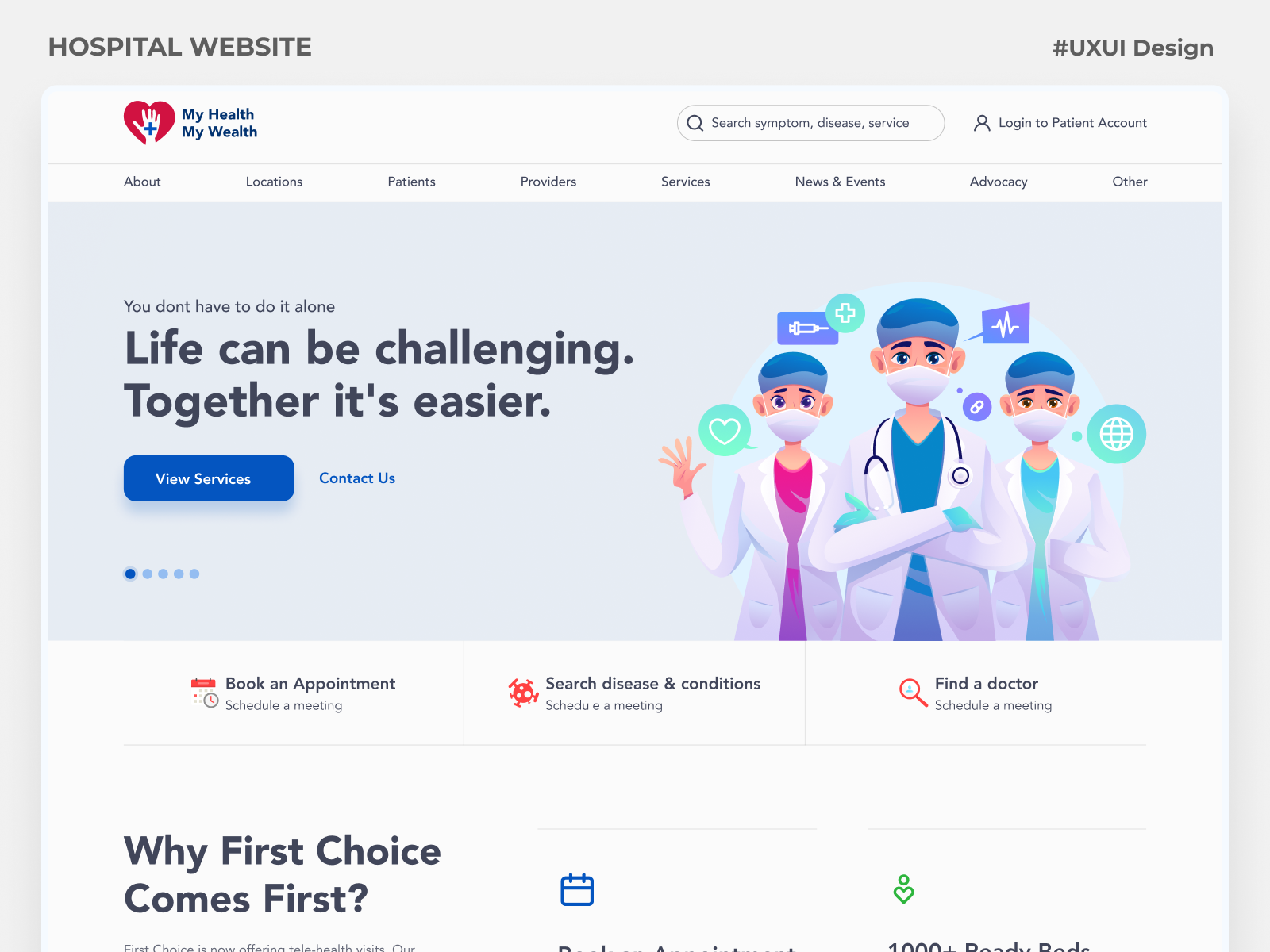The image displays a screenshot of a hospital website. 

**Top Section:**
- At the top left, the text "Hospital Website" is written in dark grey on a light grey banner. 
- On the top right, "hashtag UXUI design" is also in dark grey.

**Header:**
- The website's homepage features a white background.
- Positioned at the very top left, the text reads "My Health My Wealth" in dark blue. Adjacent to the text is a logo consisting of a red heart, a white hand, and a blue cross within the hand.
- To the right of the logo, there is a white search bar with the placeholder text "Search symptom, disease, service" in black.
- Further right, either in red or black, the text "Login to patient account" is displayed.

**Navigation Menu:**
- Below the header, there is a navigation menu with the following options from left to right: About, Locations, Patients, Providers, Services, News & Events, Advocacy, and Other.

**Main Content:**
- The main content area showcases cartoon artwork depicting three doctors. 
  - The central doctor stands with folded arms.
  - The doctor on the left is waving.
  - The doctor on the right has hands in pockets.
- All three doctors are wearing white masks and dark blue caps. Their scrubs are colored in purple, blue, and green, with white lab coats.
- The central doctor features a stethoscope.
- Surrounding the doctors are bubbles in varying colors, such as green and purple.
- To the left of the artwork, the text reads "Life can be challenging, together it's easier."

**Call to Action:**
- Below this tagline, a blue button with white text reads "View Services," and next to it, "Contact Us" is displayed.

**Additional Sections:**
- Below the call to action, further sections are visible:
  - "Book an appointment"
  - "Search diseases and conditions"
  - "Find a doctor"
- In the bottom left, there is black text reading "Why First Choice Comes First."
- Below this, there are additional sections, but they are cropped out and not fully visible. This section has a white background.